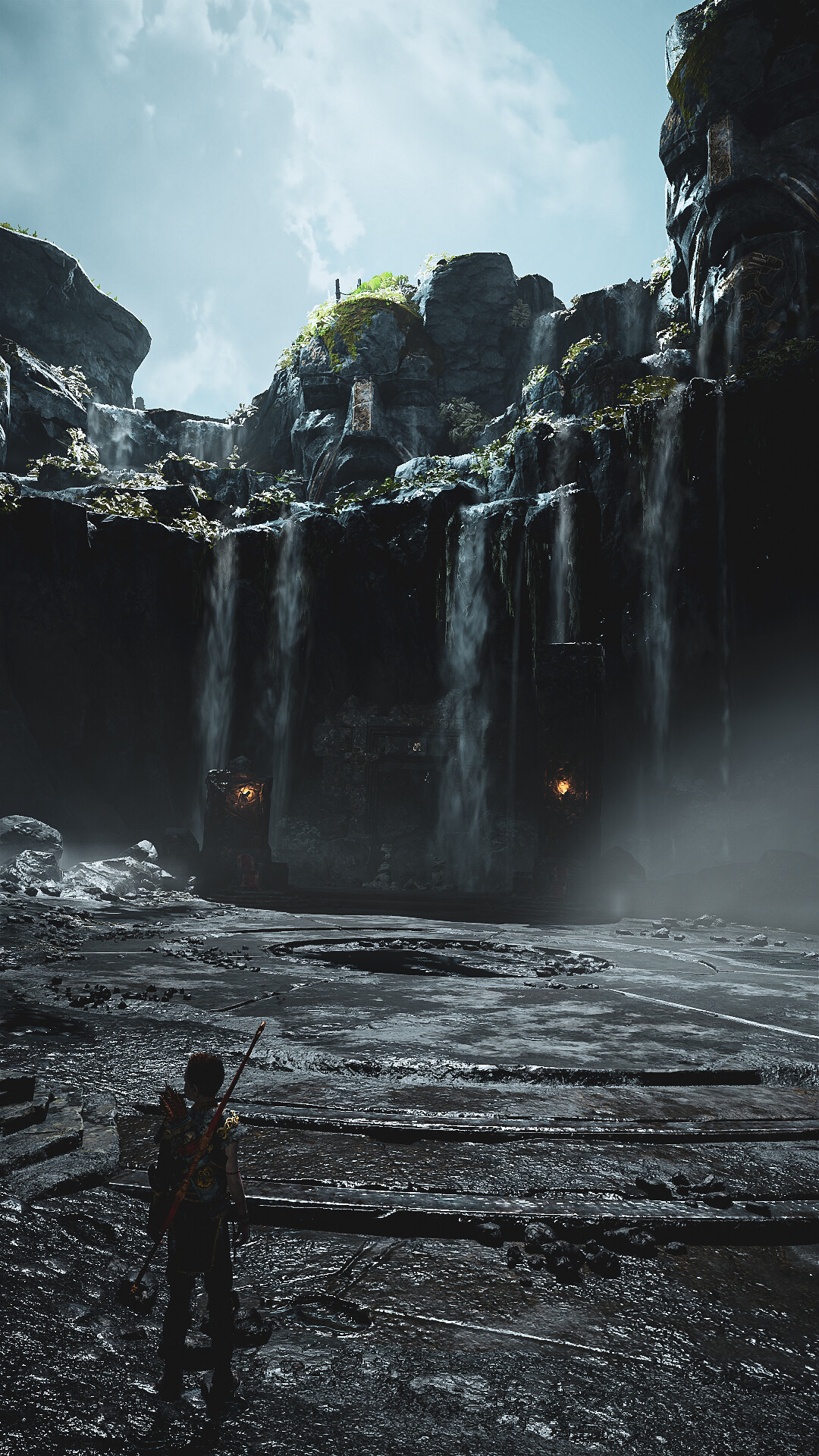The image is a hyper-realistic screenshot from a modern video game, almost indistinguishable from a photograph at first glance. The scene is set in front of a dark, rocky cliff with several small waterfalls cascading down its face, creating a dynamic and wet environment. At the bottom left corner of the image stands the main character, identifiable by their back turned towards the viewer, facing the waterfalls. The character appears armored and equipped with a bow and arrow, with the quiver visible. The ground around them is rubble-strewn and wet, but devoid of standing water directly beneath their feet, although water begins a short distance ahead. There are concrete or stone stairs to the character's left, leading up to larger, rugged boulders. The sky above is a subdued blue with fluffy clouds on the left, completing the atmospheric scene. In addition to the natural elements, small sources of light can be spotted on the wall or cliff, hinting at possible human-made structures, further detailed by what seems to be the very top of a power plant or electric generating station peeking through the rocks.